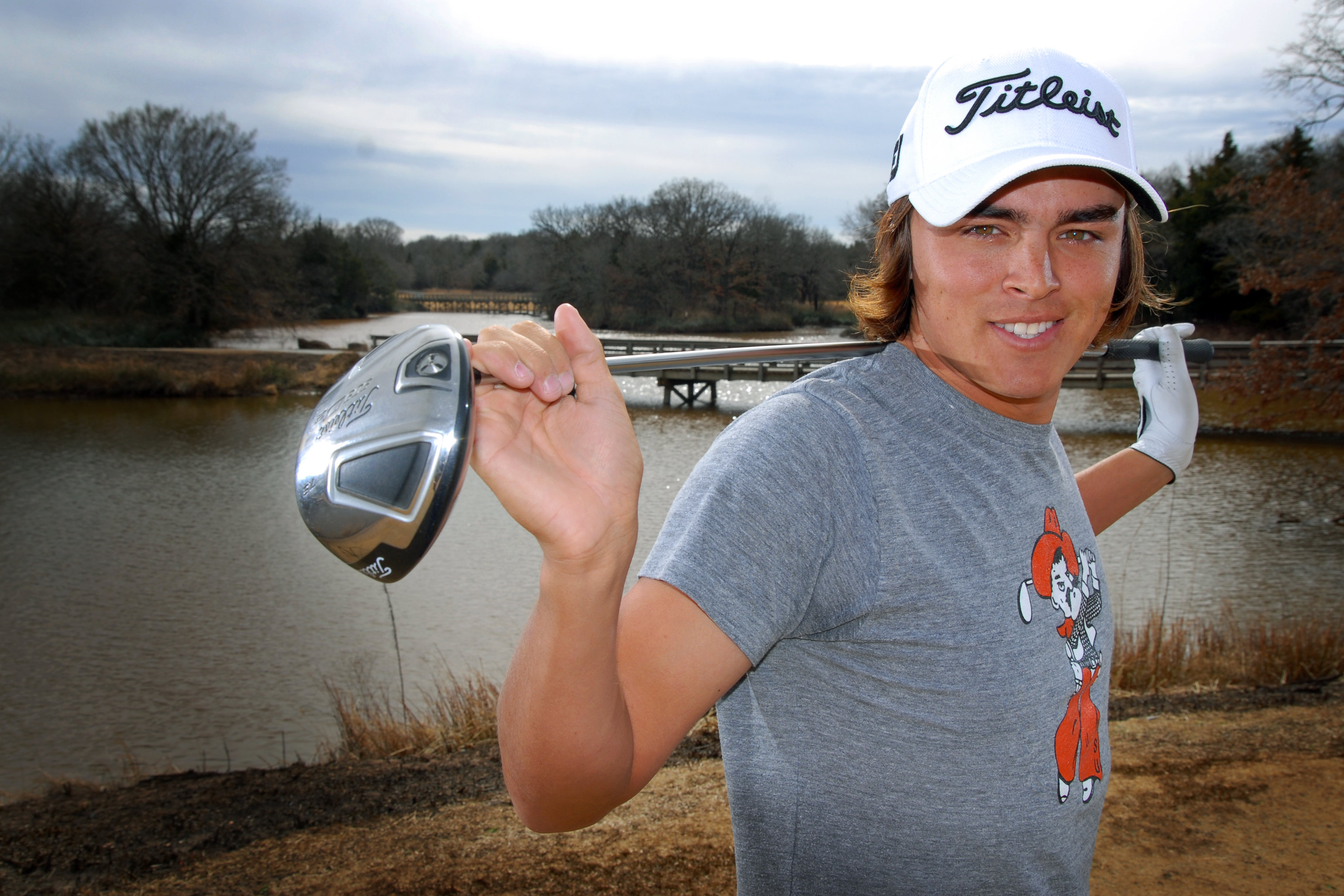In the photo, golfer Ricky Fowler is prominently posed with a driver draped across his shoulders, arms extended to hold the club at each end. Fowler sports a white baseball cap emblazoned with the Titleist logo in black cursive. On his left hand, he wears a white golf glove, leaving his right hand bare. He is dressed in a gray short-sleeve t-shirt featuring a cartoon golfer on the front. Fowler stands on mowed grass, indicative of a golf course, with a tranquil lake and scenic bridge in the background. The setting suggests it is autumn, as the area around the lake is marked by dead grass and trees with orange leaves or completely barren branches.